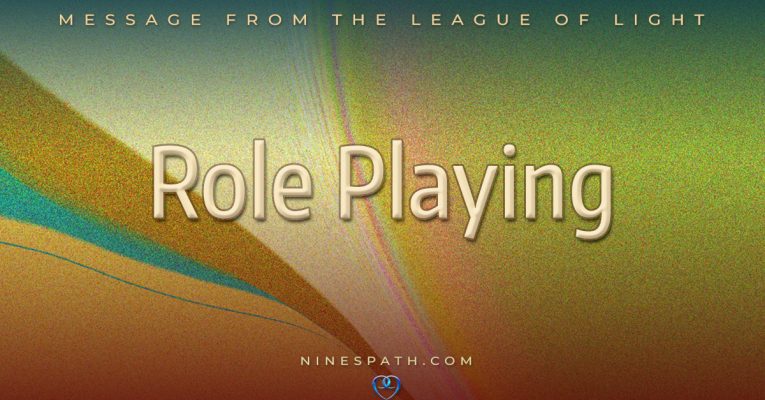This visually dynamic, horizontally-oriented advertisement card features large, centrally-positioned text that reads "Role-Playing." The background is a vibrant, swirling collage of colors including gold, blue, beige, pink, purple, yellow, orange, brown, and cream, creating a burst of energy. At the top of the card in smaller white font, the text reads "Message from the League of Light." Beneath the main heading, also in smaller white text, is the website "9spath.com," accompanied by a small blue heart design. All text elements are centrally aligned, enhancing the card’s cohesive design and highlighting "Role-Playing" as the focal point. The intricate and colorful backdrop, combined with the clear, crisp fonts, make this card both eye-catching and informative.